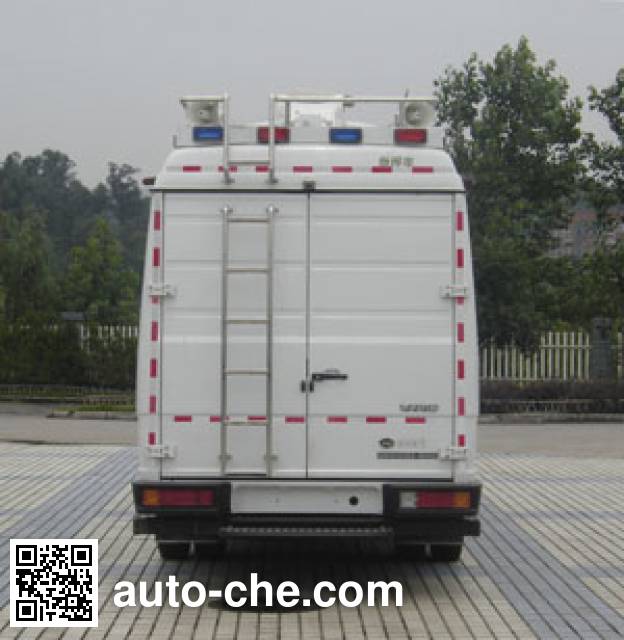This image showcases the back of a large white vehicle, most likely an ambulance due to the presence of multiple emergency lights and loudspeakers. The vehicle is parked outdoors in a parking area, which appears to be dry despite an overcast, gray sky hinting at rain. Surrounding the area, tall trees with green leaves frame the scene from the left and right, indicating a neighborhood setting with a white picket fence featuring vertical slats on the opposite side of the street. 

Centrally framed in the photograph, the vehicle's rear end is neatly detailed. It features two closed doors, a silver ladder affixed to the left side, and a door handle positioned in the middle right of the door. Distinctive red dashed lines outline the back of the vehicle in a square shape, accentuating its edges. The van boasts four alternating blue and red emergency lights arranged along the top, with spotlights situated above each end light. There are two taillights and a black bumper at the bottom. Additionally, a barcode is visible in the lower-left corner of the vehicle along with the website "auto-chi.com" printed in white letters.